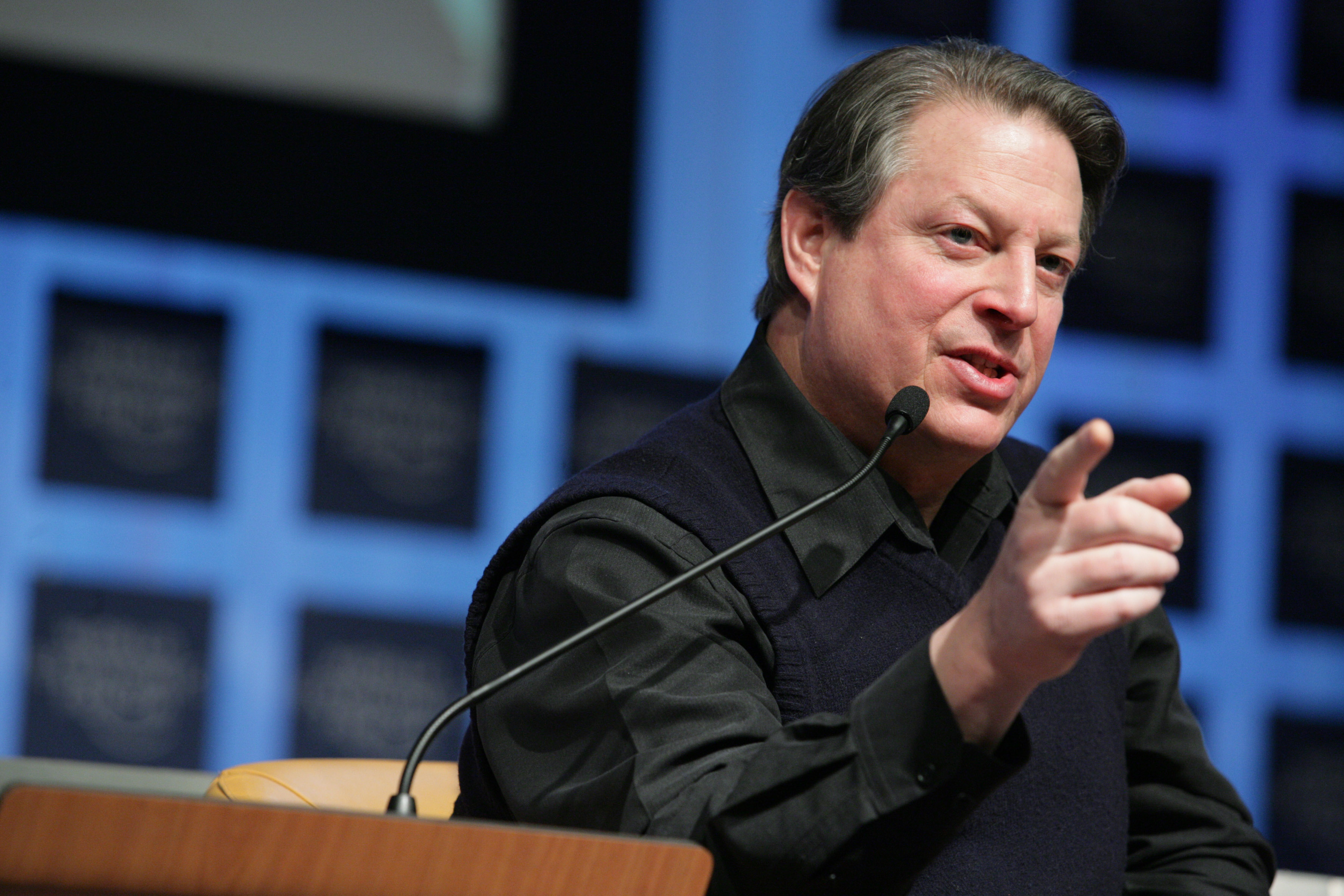The photograph captures an older man in the midst of giving a presentation on stage. He is seated in a yellow upholstered chair, visible from the stomach upwards, and dressed in a black long-sleeved button-up shirt with the top button undone, paired with a black V-neck sweater vest. With graying black hair and dark eyes, he faces the right side of the image and points forward, possibly addressing a question. Adjacent to him, a light brown podium holds a stand microphone positioned close to his mouth. Behind him, a light blue background features multiple black squares, one notably larger but partially cropped by the photo's frame. The composition suggests a professional setting, likely a conference or panel discussion.